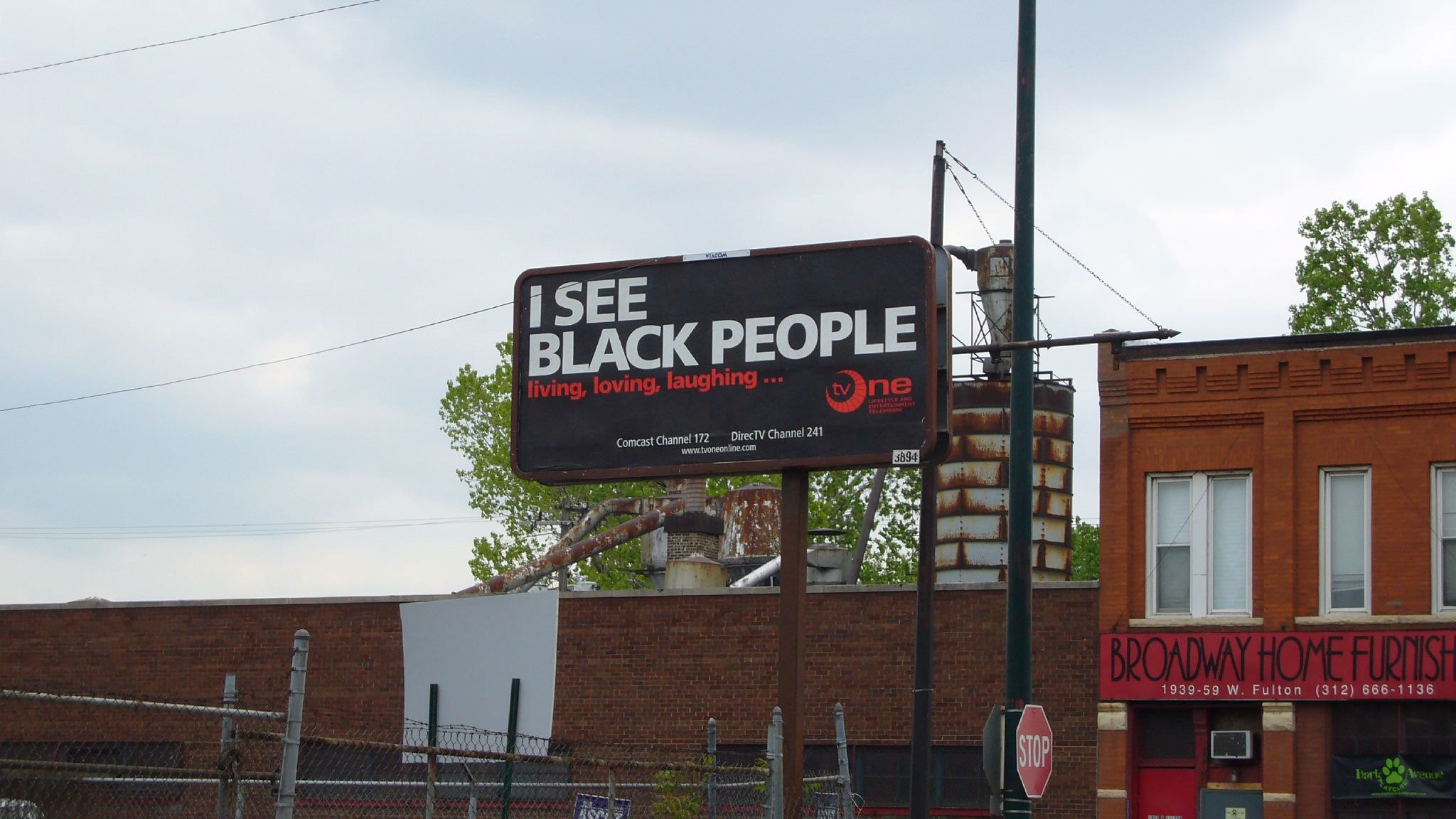This color photograph, taken outdoors, captures a section of a city street featuring two brick buildings and a billboard. On the right-hand side, there is a two-story red brick building adorned with large windows on its second floor. The building prominently displays a burgundy sign with black font that reads "Broadway Home Furnish," alongside the address "1939-59 W Fulton" and phone number "(312) 666-1136" in white font. Adjacent to this structure, a metal stop sign is affixed to a power pole.

To the left of the brick building, a large billboard with a black background features the white text "I see black people," followed by the red text "living, loving, laughing." The billboard also includes a crescent moon graphic in red. Below the billboard, a shorter, single-story brick building is visible, which has a white smokestack that appears rusted. In front of these buildings, a chain-link metal fence adds to the urban landscape.